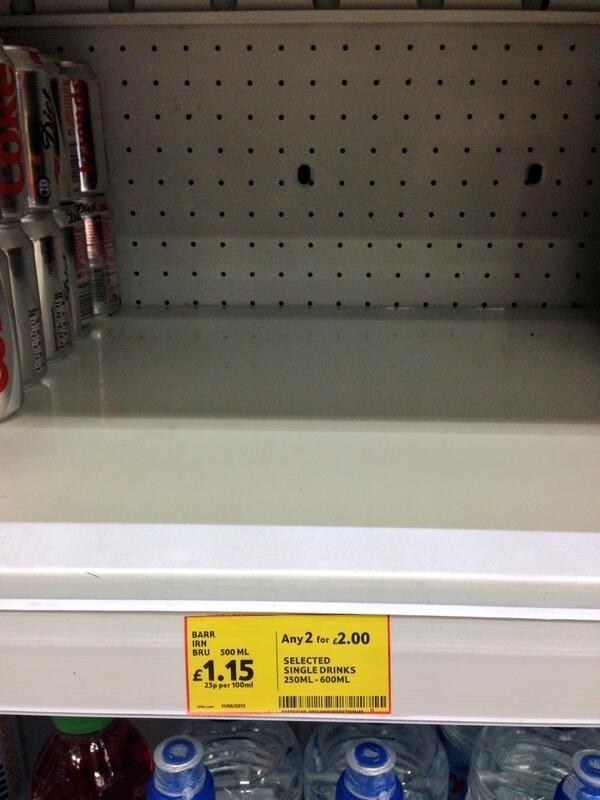In a retail store, a white wall provides a clean backdrop, complemented by a distinctive checkered ceiling dotted with small designs. A clear piece of glass features a neat white bar across it, which holds a prominent yellow sticker. The sticker advertises a discount: "$1.15 each, or any two Iron Brew 500ml for $2. Selected single drinks range from 250ml to 600ml." Below the glass, clear plastic bottles are neatly arranged, most with blue lids, while one dark colored bottle with a green lid stands out to the left. For those interested in beading supplies and design ideas, visit www.beadaholique.com.